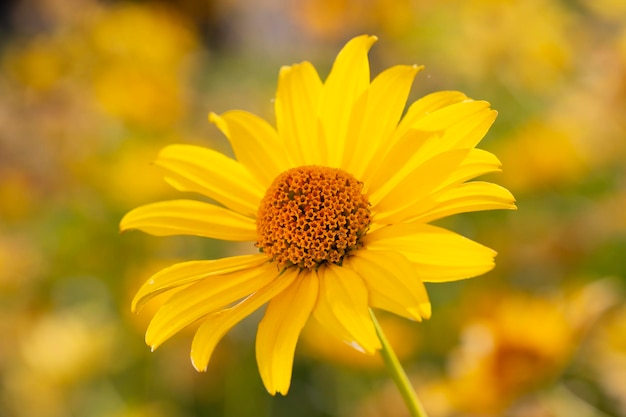The photograph captures a vibrant yellow flower in sharp focus, highlighted by its thin oblong-shaped petals that surround a central semicircle adorned with star-shaped filaments. The core of the flower displays a darker golden-yellow hue, contrasting with the bright yellow of the petals. This prominent flower is attached to a thick, smooth green stem that extends out of the frame at the center of the image. The background, rendered with a bokeh effect, subtly reveals a field filled with similar yellow flowers and green plants in an outdoor setting, accentuating the photograph's natural and colorful ambiance. The image, characterized by its high-definition clarity and rectangular shape—where the width is twice its height—places emphasis on the beautifully detailed flower in the foreground while softly blurring the surrounding floral scenery.